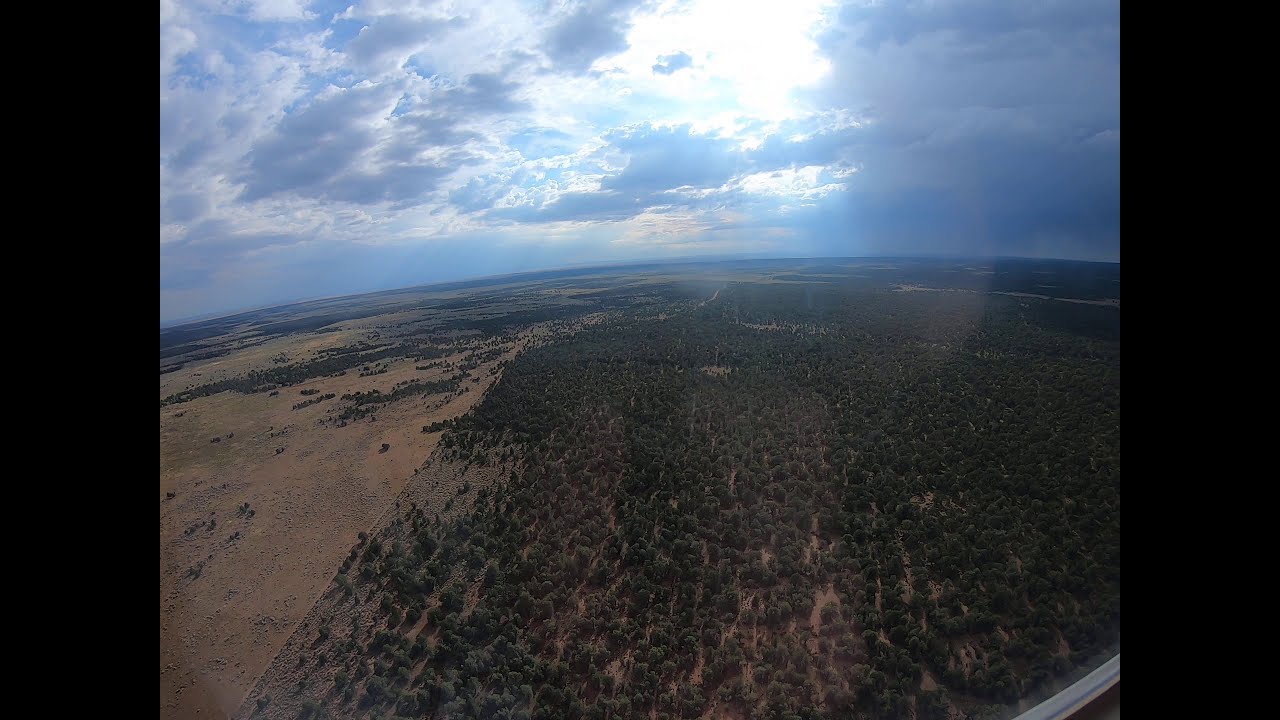This detailed photograph captures a sprawling landscape viewed from above, likely taken from a drone or a low-flying aircraft such as a helicopter or a Cessna. The image, presented in a landscape orientation, features vertical black rectangular frames on both the left and right sides, adding a striking border to the scene.

Dominating the lower portion of the image is a dense patchwork of scruffy green vegetation, interspersed with clusters of small trees and bushes. To the left, a raw expanse of red dirt indicates a barren area with no vegetation, likely marking a property line. A small road can be seen trailing into the distance along this border, emphasizing the contrast between the green expanse and the open, brown land. This road appears to fade into the horizon, where the flat landscape stretches endlessly without any mountains in sight.

The sky above is a tableau of varying shades of gray clouds, darker to the right and left, with a brighter section in the middle where the sun is valiantly attempting to break through. Its light creates a dramatic effect, illuminating parts of the landscape while casting deeper shadows in others. The photograph does not feature any people, vehicles, or text, maintaining the pristine natural beauty of the scene.

Overall, the image epitomizes photographic realism, capturing the intricate details of the earth's surface and sky in a true-to-life representation.